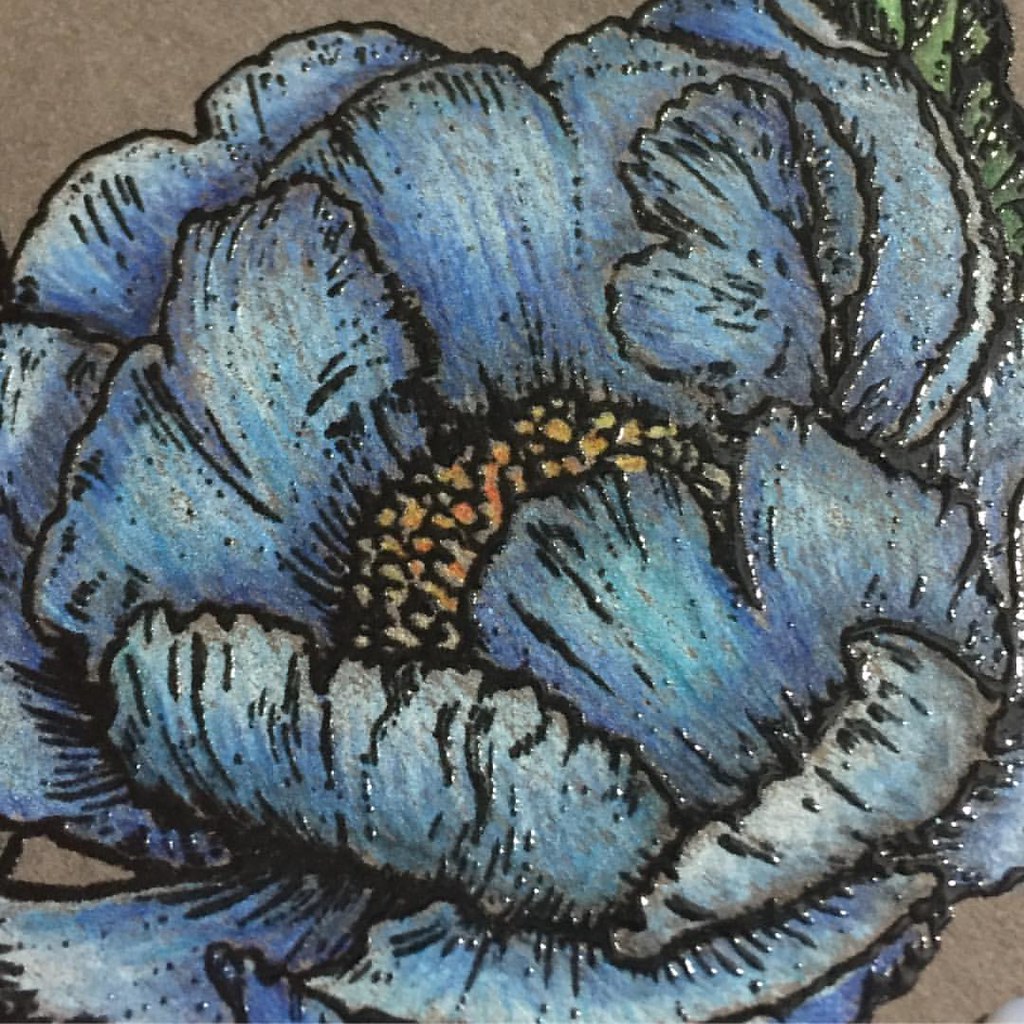In the middle of a textured, cardboard-like background, a captivating blue flower prominently stands out. The flower is composed of numerous petals that radiate outward and upward, each exhibiting intricate details. Every petal is infused with subtle shades of brown and meticulously outlined with striking black edges, further accented by delicate black markings. At the very heart of the flower, a vibrant yellow center draws the eye, with additional yellow accents scattered across some petals, adding depth and contrast to the composition. This intricate flower arrangement, encased in an earthy, minimalistic background, beautifully highlights the contrast and harmony of its colors.